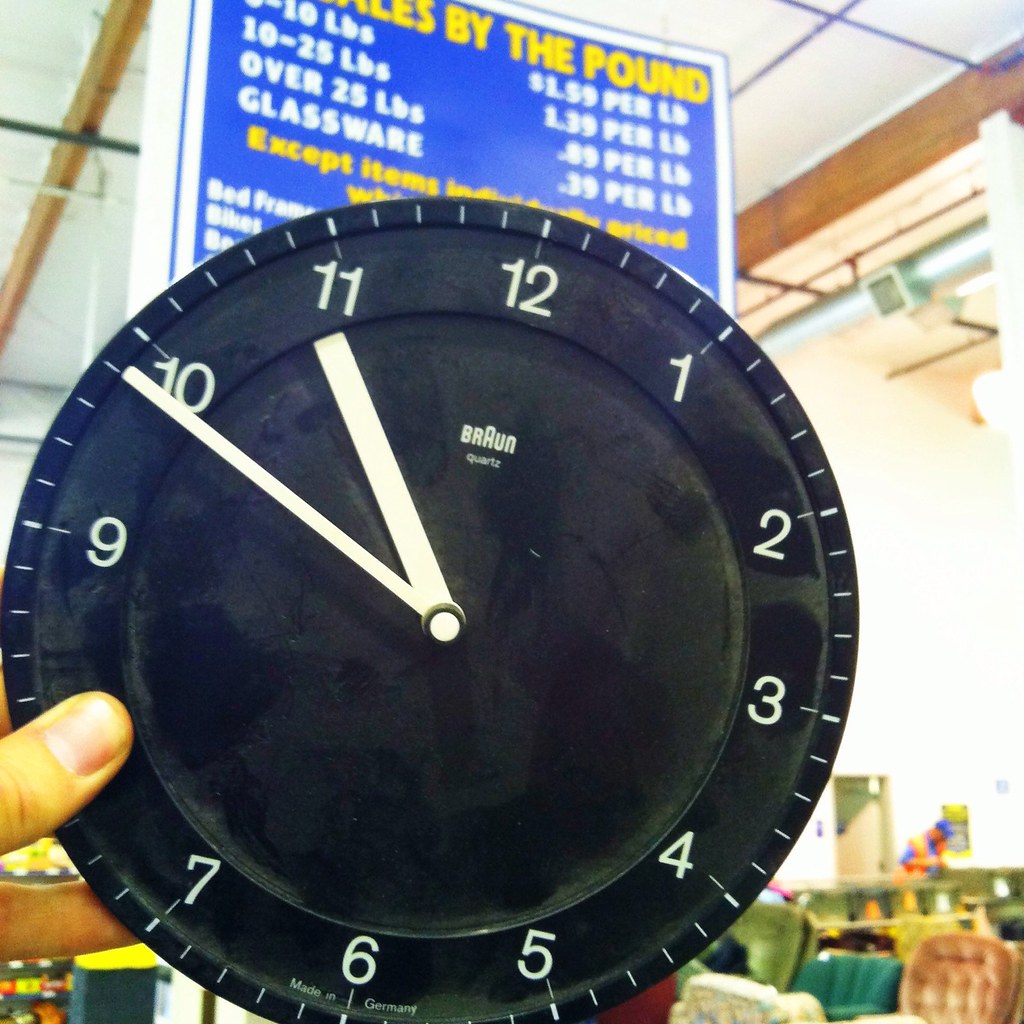This image features a close-up of a black, round clock with a white trim. The clock face displays white numbers from 1 to 12, with smaller hash marks denoting individual minutes around the perimeter. The hour hand is near the 11 while the minute hand is close to the 10. Below the 12, the brand name "Braun" is prominently displayed in white, with a larger 'A' in the center, followed by "Quartz." Additional text at the bottom by the 6 reads "Made in Germany." A person is holding the clock, likely male with an olive complexion, gripping it with their thumb and forefinger from either the left or right side. The background suggests a department store setting, with visible store signs, furniture of various colors (dark green, red, olive green, and white), and shelving units. Above the clock, a large blue sign with yellow text reads, "by the pound," among other details partially obscured by the clock. The overhead ceiling appears white with light brown beams.